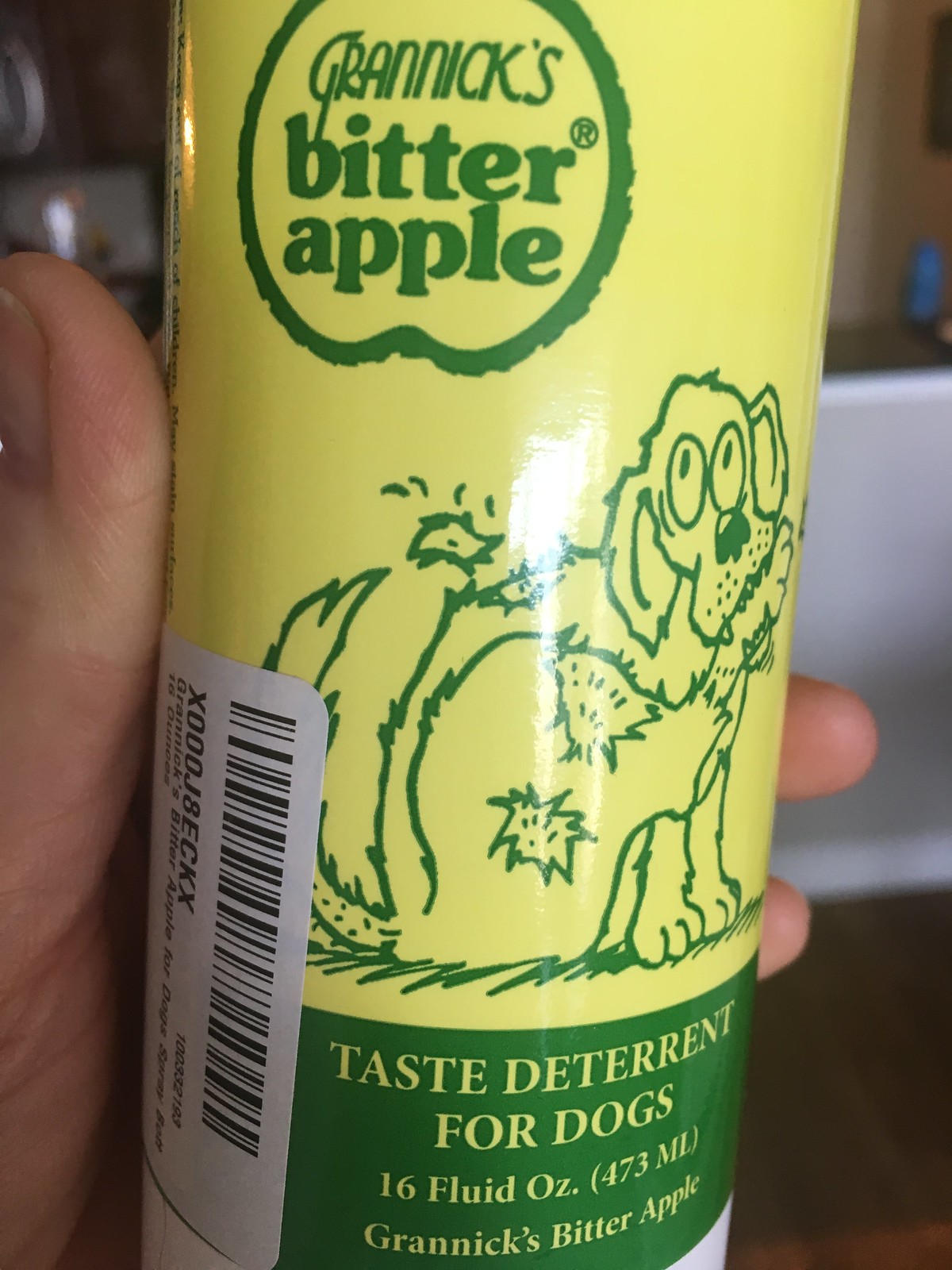The image features a bright yellow plastic bottle with a light green label, identified as a product from Granick’s Bitter Apple, specifically labeled as a taste deterrent for dogs. The label prominently displays the brand name “Granick’s Bitter Apple” in green text, encased within the outline of a green apple. Below the brand name, there is a cartoon-like sketch of a dog, resembling a golden retriever, depicted chewing on its foot with patches of fur missing. The label further states the bottle's capacity as "16 fluid ounces (473 milliliters)." There is a white barcode sticker on the left-hand side with the code "X000J83CKX." The bottle is being held by a hand emerging from the left side of the image, with the thumb raised vertically and fingers wrapped around the bottle. The background shows a wooden floor beneath a white shelf, with some kitchen utensils visible in the top left corner.